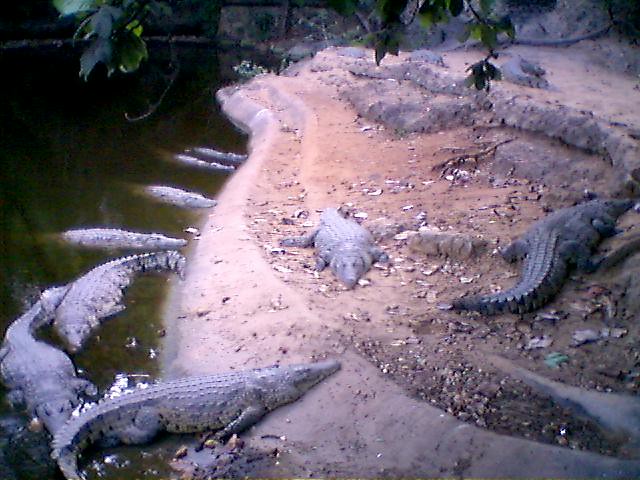This detailed photograph captures a bustling scene of either alligators or crocodiles congregating in a murky, swamp-like area. Towards the bottom and left of the image, many of these reptiles are partly submerged in the water, which is a cloudy brownish-green color, indicative of its muddy and moss-infused nature. Some of the creatures are lounging on the sand or a dirt island that emerges from the water. 

The right side of the image features a rock area strewn with leaves and dirt, which seems to possess two levels – one directly above the water and another higher up towards the upper right of the image, giving these reptiles space to climb and bask. A dark gray alligator, the darkest among them, is prominently seen climbing onto this rocky incline in the foreground, while others of varying lighter shades are scattered about.

The top part of the image reveals green foliage hanging down, providing a lush backdrop to the scene. The atmosphere appears dim, suggesting an overcast day. This snapshot encapsulates a typical swamp habitat, with these reptiles, possibly a family, lounging in their natural environment, both in the water and on the land, leisurely basking or navigating their surroundings.